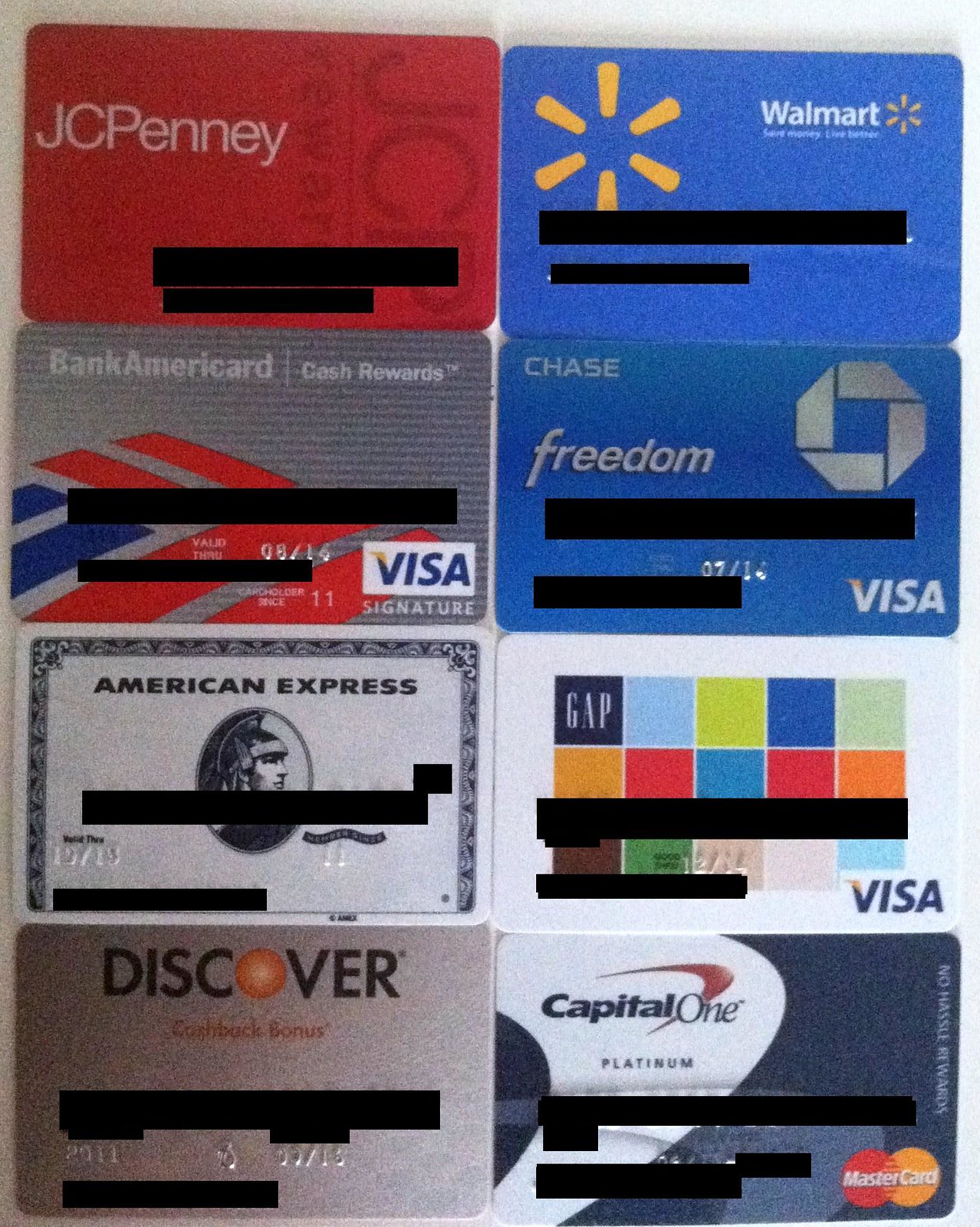This is a photograph displaying a variety of credit and store cards, with black stickers concealing the card numbers and names for privacy. In the top left corner is a red JCPenney card with white lettering. To its right is a blue Walmart card adorned with a yellow star logo. Below the JCPenney card is a Bank of America Cash Rewards card, characterized by gray with red and blue chevrons, which features the Visa logo. Adjacent to that is a blue Chase Freedom Visa card marked with "0714". Moving further right, there's a silver American Express card stamped with "1913", although it's hard to read. Next to the American Express is a blue Gap Visa card, featuring a multicolored, three-block-high design. Below the Bank of America card sits a Discover cashback bonus card, which is almost gray in color. Finally, on the bottom right is a gray Capital One Platinum MasterCard, distinguished by its white and red "swish" logos. The collection includes cards from various types: Visa, MasterCard, Discover, and American Express, alongside store-specific cards from JCPenney, Walmart, and Gap.